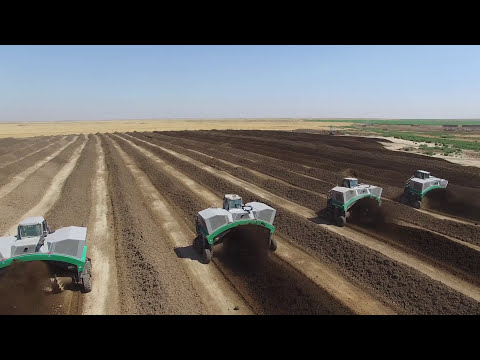The photograph captures an expansive farm scene viewed from above, showcasing four heavy agricultural machines meticulously working in tandem to create neatly aligned rows in the soil. These machines, identifiable by their white and green coloration and open central sections flanked by four wheels on either side, appear to be either planting seeds or preparing the soil. The field, stretching nearly half a mile into the distance, is composed of alternating dark brown furrows— indicative of where the machines have already passed—and lighter brown areas awaiting treatment. The scene includes a backdrop of light beige soil and patches of green grass on both the left and right edges, further accentuated by a vivid blue sky that spans the top quarter of the image. Each machine has a visible operator in the cockpit, closely following the others along their designated rows. The clarity and brightness of the image suggest it was taken on a clear, sunny day, with natural light illuminating every detail. The overall composition is elegantly framed by a black border at both the top and the bottom, highlighting the large, open field as the central focus.